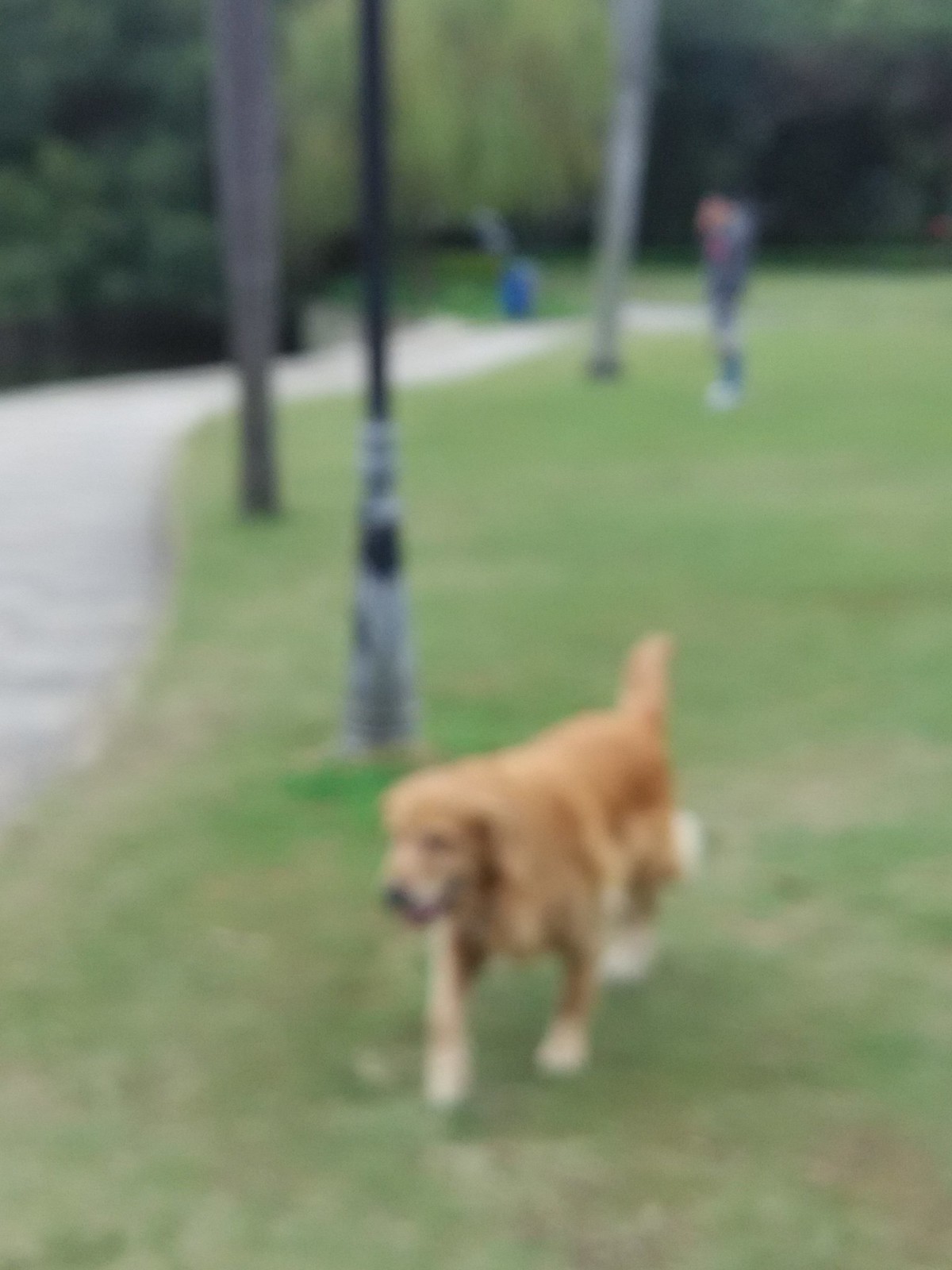The image depicts an outdoor scene with a low-resolution, blurry quality. At the bottom center of the image, a light brown dog with white paws and a black nose stands on a grassy field. Towards the top right, a person is visible, also standing on the grass. The background is adorned with trees. Despite the poor image quality, the details of the dog and the outdoor setting are discernible.